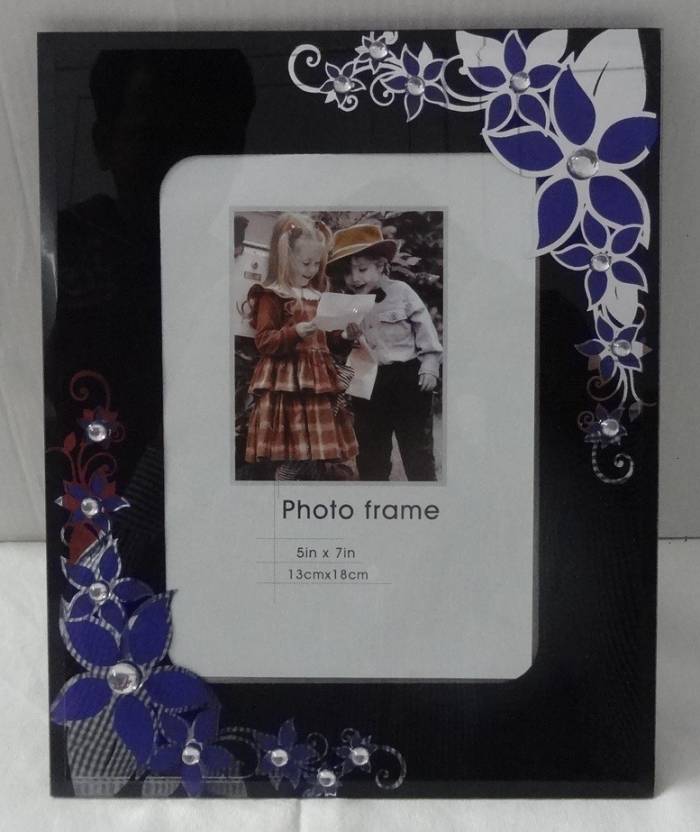The image captures a rectangular photo frame set against a gray background, which appears to be a floor meeting a wall. The frame itself is predominantly black and features intricate decorative details, including blue and white flowers accented by silver designs at the top right and blue and red flowers with similar accents at the bottom left. These flowers have rhinestone centers that add a touch of sparkle. The shiny black frame also shows a faint reflection of a person's face, suggesting its glossiness.

Within the frame, there's a beige square that reads "Photo Frame 5 inches by 7 inches, 13 centimeters by 18 centimeters" in black letters. The frame contains a stock photo of two children. The little girl, who has blonde hair styled in pigtails, is dressed in a red and white pleated dress and holds a piece of paper. Next to her, a boy wears a hat, a button-down shirt, and black pants; he holds a folded paper in his hand. The children appear to be reading letters, contributing to a sentimental and nostalgic atmosphere.